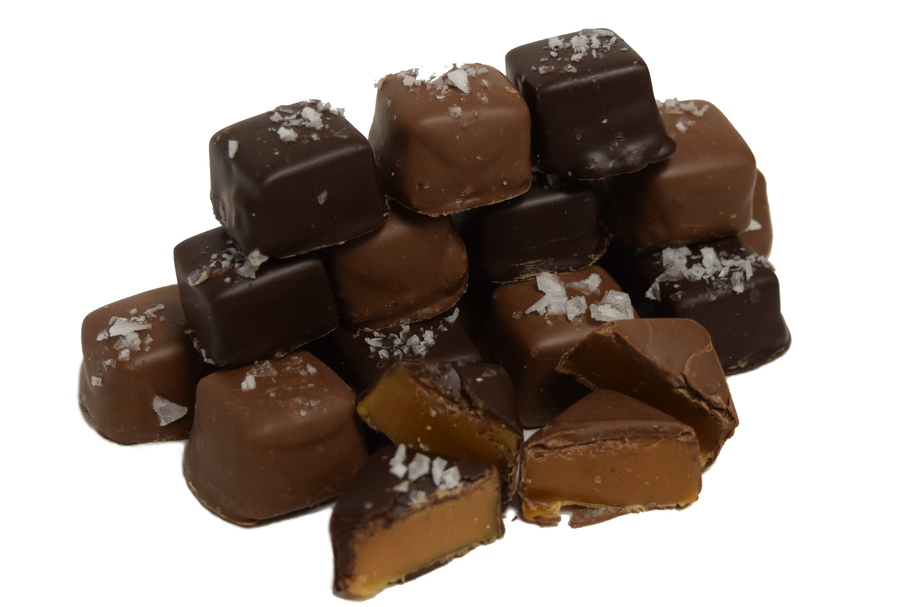The photograph displays an intricate arrangement of assorted chocolates stacked to form a small, wall-like structure against a stark white background. These chocolates, predominantly square with some rounded edges, are piled three rows high and showcase a variety of textures and colors. The assortment includes both milk and dark chocolate pieces, some of which are cut open to reveal rich caramel or fudge fillings. The surfaces of these chocolates are generously sprinkled with what appears to be shavings of coconut and possibly sea salt, adding a tactile, delicate touch to the overall presentation. The meticulous stacking and decorative elements suggest a sophisticated, almost artisanal quality reminiscent of premium boxed candies, evoking brands like Russell Stover.